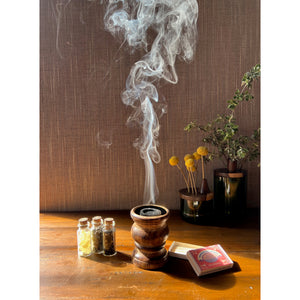In a tranquil corner of a room, three small bottles with rubber caps are neatly arranged side-by-side on a wooden floor. The leftmost bottle contains a bright yellow item, accentuated by sunlight streaming in from the left, while the other two bottles appear to hold a dark, possibly black substance. At the center of this serene setup is a copper-colored cup, likely an incense holder, with a black core and a smaller inner circle, from which delicate spirals of smoke gently rise and disperse. To the right, a closed matchbox lies next to the cup. In the background, against a dark brown wooden wall, stand two potted plants: a shorter one with yellow flowers on the left and a taller one with green foliage on the right. The scene exudes a peaceful ambiance, suggesting a space for meditation or calm reflection.